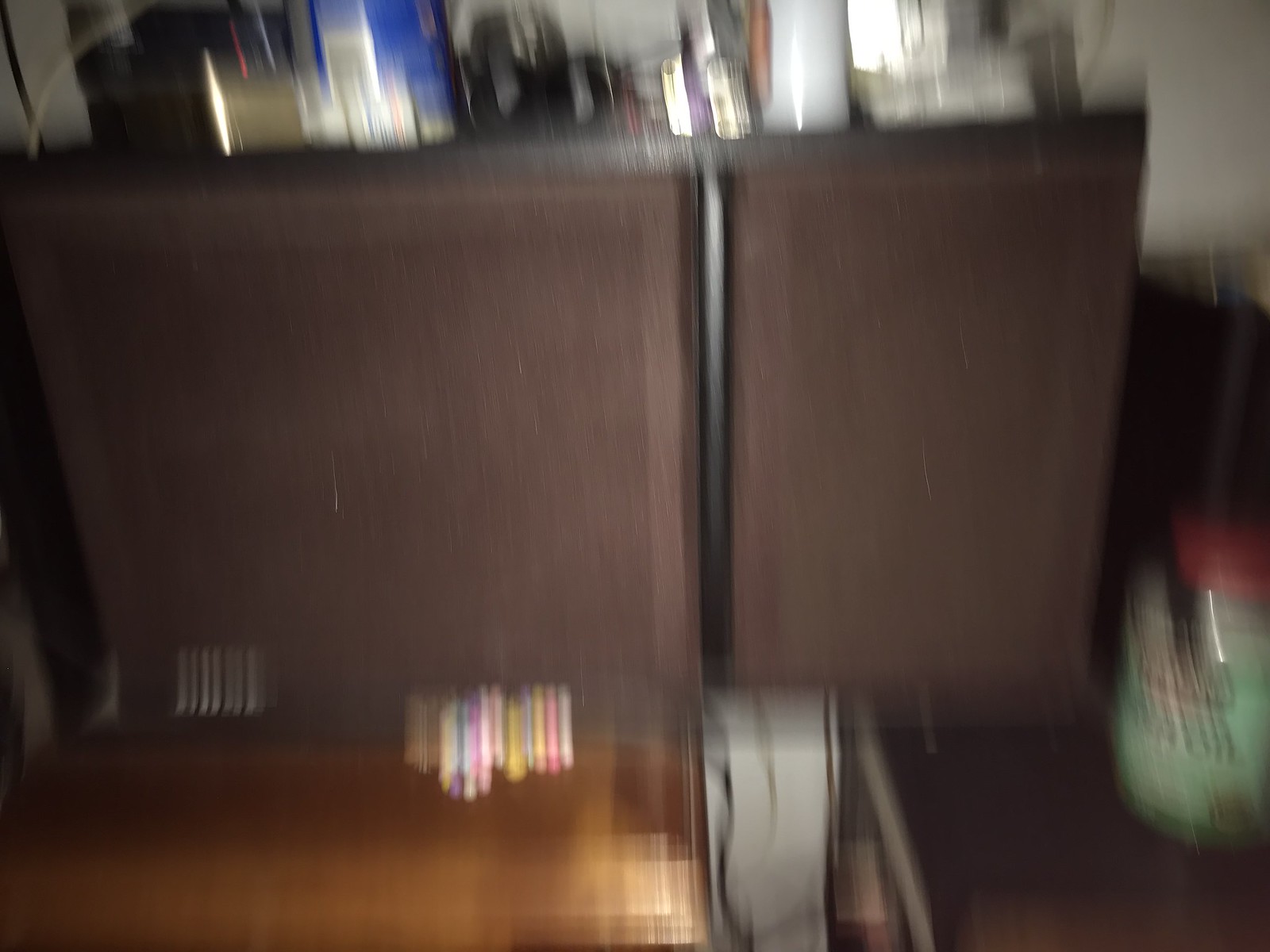A blurry photograph depicts a brown cabinet adorned with various objects including blue, white, and silver items. The image is marred by vertical streaks. The scene is set in a room where a section of the white wall and a portion of a window frame, likely illuminated, are visible in the background. On the floor to the right of the cabinet, there is a large, light green container with indistinct writing and a red lid. To the left in front of the cabinet, either on the floor or a small light brown table, several markers or crayons are scattered.